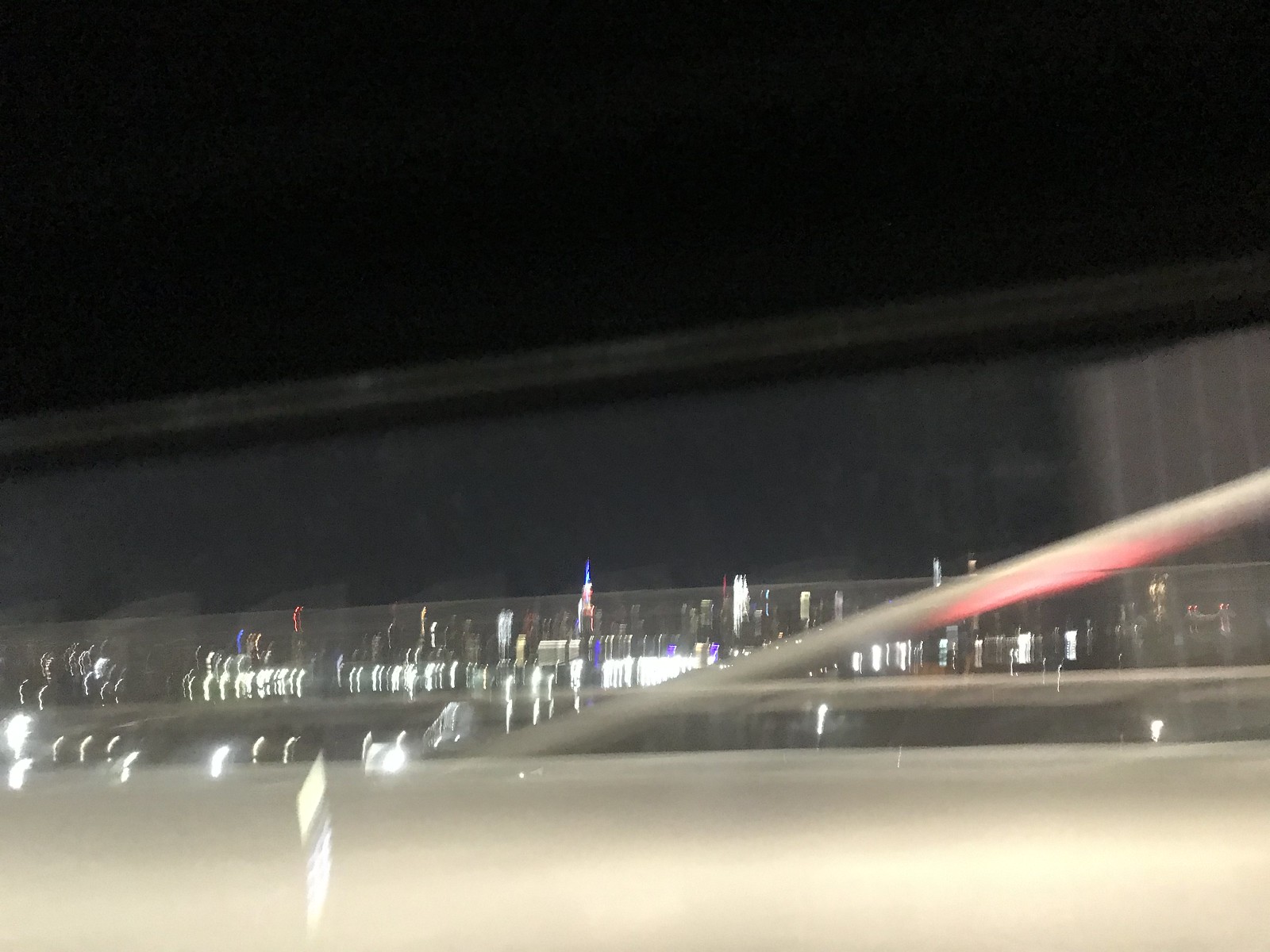A blurry nighttime image showcasing an urban landscape teeming with lights. In the foreground, a wall is visible with a pipe extending diagonally from the lower left to the upper right. The background is dominated by a tall tower adorned with white lights along its sides and topped with a blue light. The setting appears to be captured from a bridge, offering a vantage point over a cityscape filled with various buildings and lights. Despite the image's lack of clarity, it conveys the bustling vibrancy of an illuminated city under a black sky, with a myriad of lights from structures scattered across the horizon.